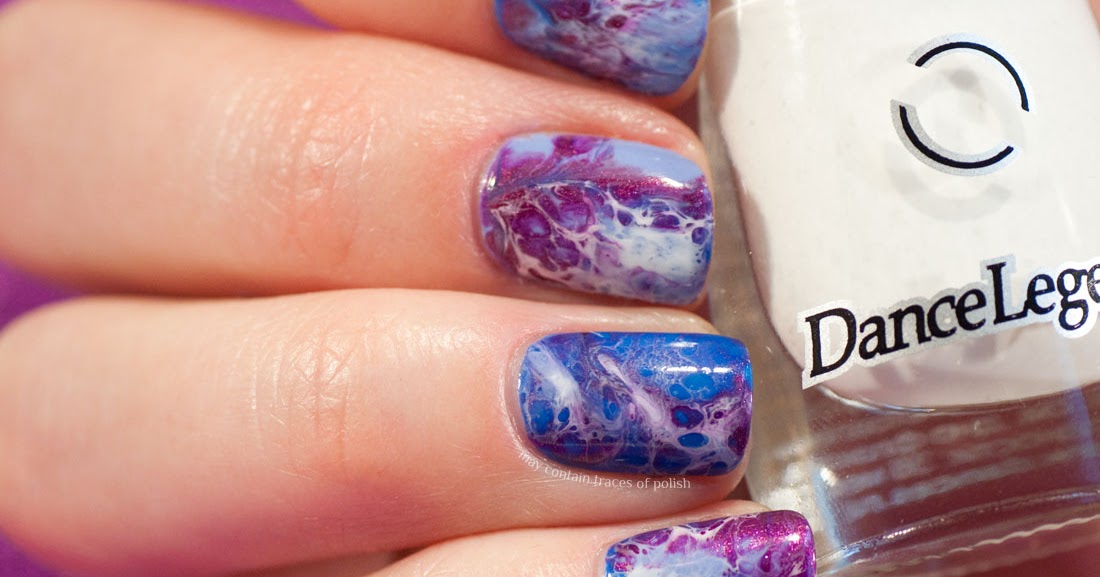This close-up photo showcases a pair of well-manicured female fingernails, emerging from the left side of the frame, primarily featuring the middle and fourth fingers, with partial visibility of the index and pinky fingers. The skin appears pale and the fingers are somewhat chubby. The fingernail polish is intricate and vibrant, presenting a marbled pattern of medium blue, purple, white, and pale gray hues, reminiscent of a cosmic or space-like theme. Tiny sparkles add to the elaborate design, making the nails resemble beautifully polished stones. The fingers are delicately holding a clear glass bottle of white nail polish, partially revealing the brand name "Dance Legend," though some text is cut off. Additionally, faint text on one of the nails reads "May contain traces of polish." The overall composition highlights the ornate beauty and detailed artistry of the nail design.